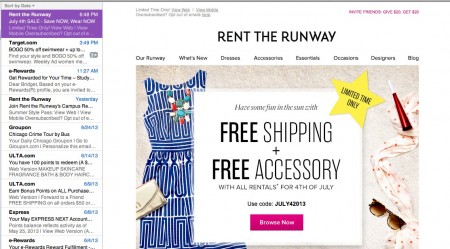Screenshot of an email service interface displaying an opened email from Rent the Runway:

The left pane showcases a list of emails, most of which are unread and denoted in bold font. The topmost email from Rent the Runway has been read, indicated by its normal font and highlighted in purple.

In the right pane, the email preview reveals a vibrant marketing message from Rent the Runway, featuring a promotional banner that reads, "Have some fun in the sun with free shipping and a free accessory with all rentals for the 4th of July." The email advertises a limited-time sale, providing a special discount code. Additionally, it offers a "Browse Now" option for immediate shopping.

The email also highlights various categories available on the Rent the Runway website, such as "Our Runway," "What's New," "Dresses," "Accessories," "Essentials," "Occasions," "Designers," and a "Blog." There's a referral incentive displayed, stating, "Invite Friends: Give $20, Get $25," although the text appears slightly blurry.